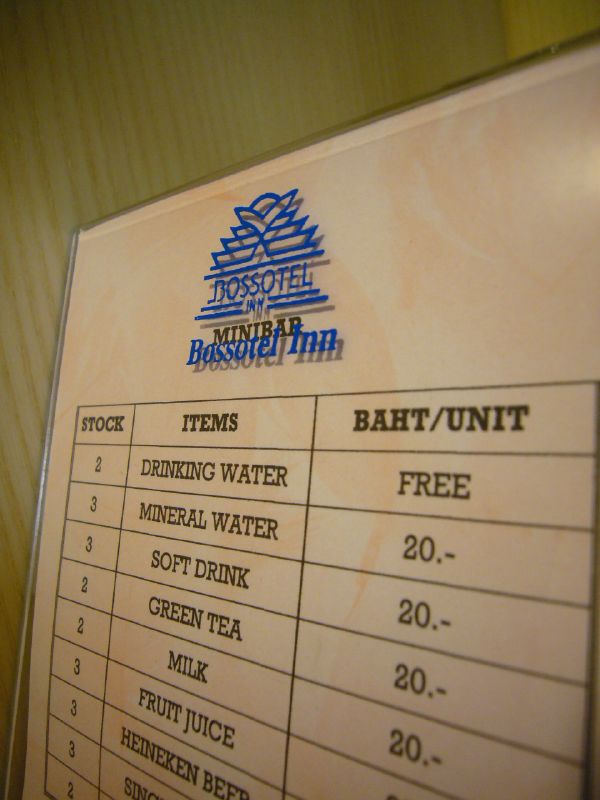The image features a detailed price list for a minibar at a hotel named Basotel Inn. The sign, which appears to be lying on a light tan or creamy white surface with abstract light orange swirls, has a blue design at the top with the text "Minibar Basotel Inn." The menu is organized in a tabular format with columns labeled "Stock," "Items," and "BHT/Unit." The listed items are beverages, with the first item being drinking water, which is available for free. Other drinks include mineral water, soft drinks, green tea, milk, and fruit juice, each priced at 20 baht per unit. There is also Heineken beer, but its price is not visible. The stock numbers for each item range from two to three units. The sign resembles a large menu typically displayed in a hotel lobby to inform guests about available minibar items.